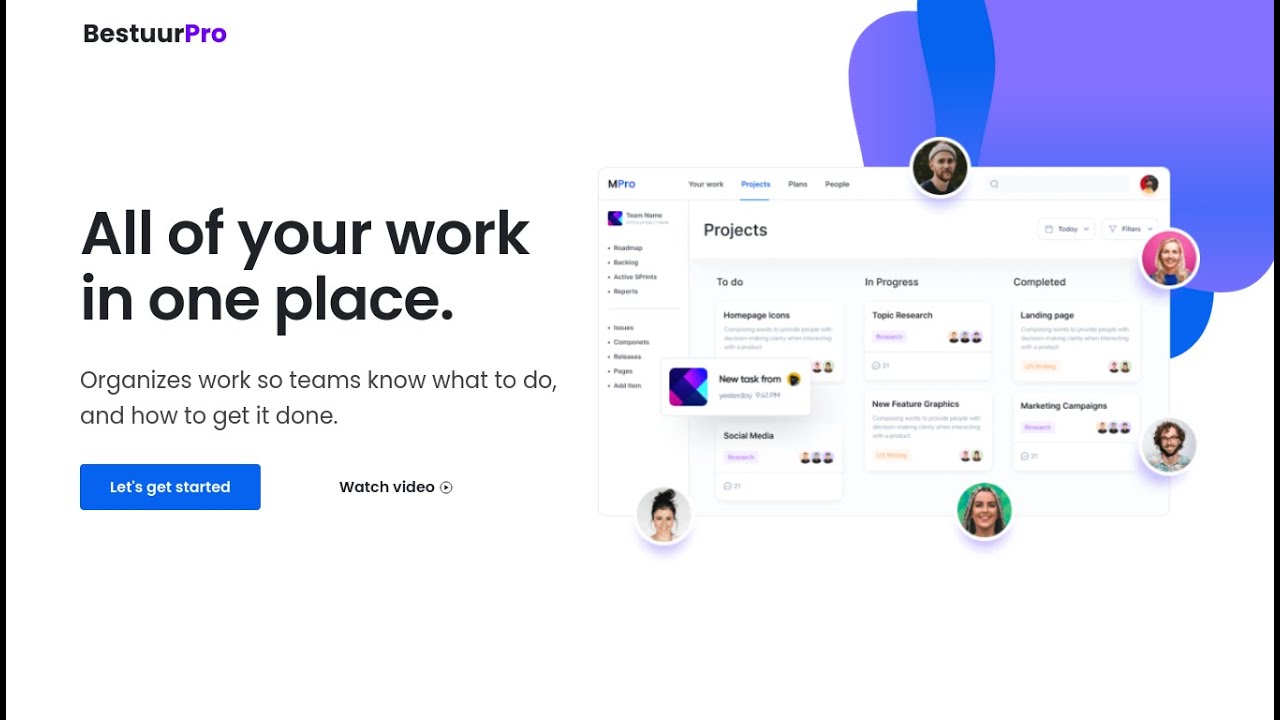The image depicts the homepage of the website "BESTURPRO." The word "BESTUR" appears in black, while "PRO" is highlighted in purple. The background is predominantly white, providing a clean and minimalist aesthetic. 

The page is designed to offer a comprehensive workspace where teams can manage and organize their tasks. Prominently featured is a blue button with white text that reads "Let's Get Started," inviting users to begin using the platform. Adjacent to this is a link, accompanied by a right arrow, that encourages users to "Watch Videos."

The main navigation includes tabs labeled "Projects," "To Do," "In Progress," and "Completed," effectively segmenting different stages of work. Additional icons direct users to various sections such as Home, Topics, Research, Landing Pages, Market Campaigns, New Features and Graphics, New Tracks, and Social Media Tasks.

The color palette of the website is notably diverse, incorporating shades of white, black, purple, blue, pink, green, gray, yellow, as well as natural hair colors like brown, blonde, and black. 

A black vertical strip runs along the left side of the layout, adding a sleek, contrasting element to the design.